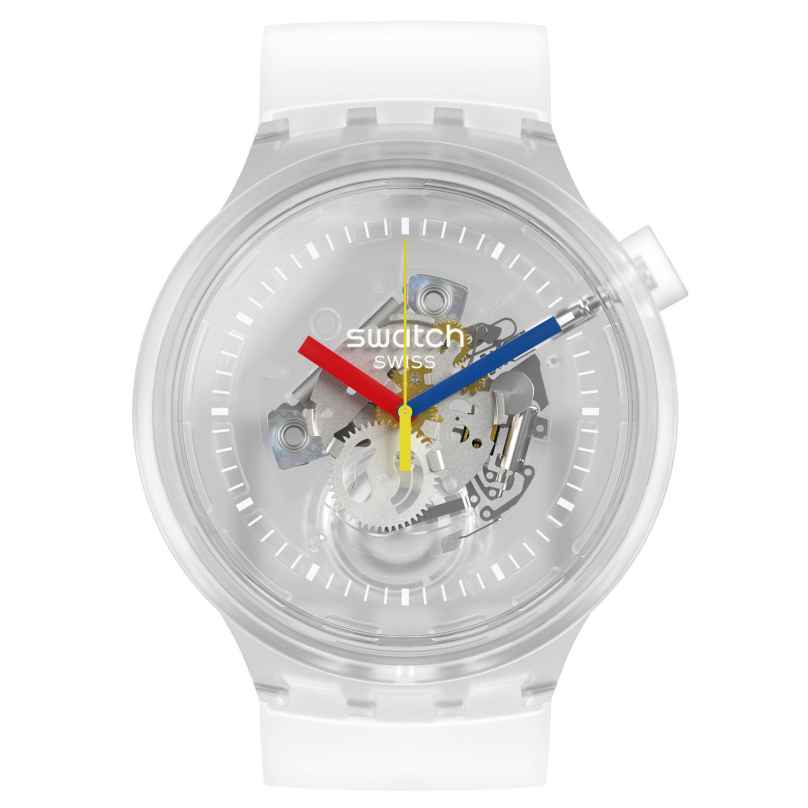The image depicts a close-up view of a Swatch watch face against a completely white background. Only the very top and bottom parts of the clear or white band are visible, as the majority of the image is focused on the watch face itself. The watch face features a light gray background, with white tick marks representing the hours encircling the dial. Prominently displayed in the center are the words "Swatch" in white letters and "SWISS" in smaller all-cap letters beneath. The hour hand is a slender red rectangle, pointing to the 10 o'clock position, while the minute hand is longer, blue, and points towards 2 o'clock, ending in a silver tip. The second hand is a thin yellow line, positioned at the 12 o'clock mark. The transparent cover reveals the intricate inner workings, showcasing a mix of silver, clear, and gold-colored gears and mechanisms, which add an interesting depth to the design. The watch's clear and white casing, along with the visible transparent winding mechanism near the top right, emphasizes its modern and minimalistic aesthetic.